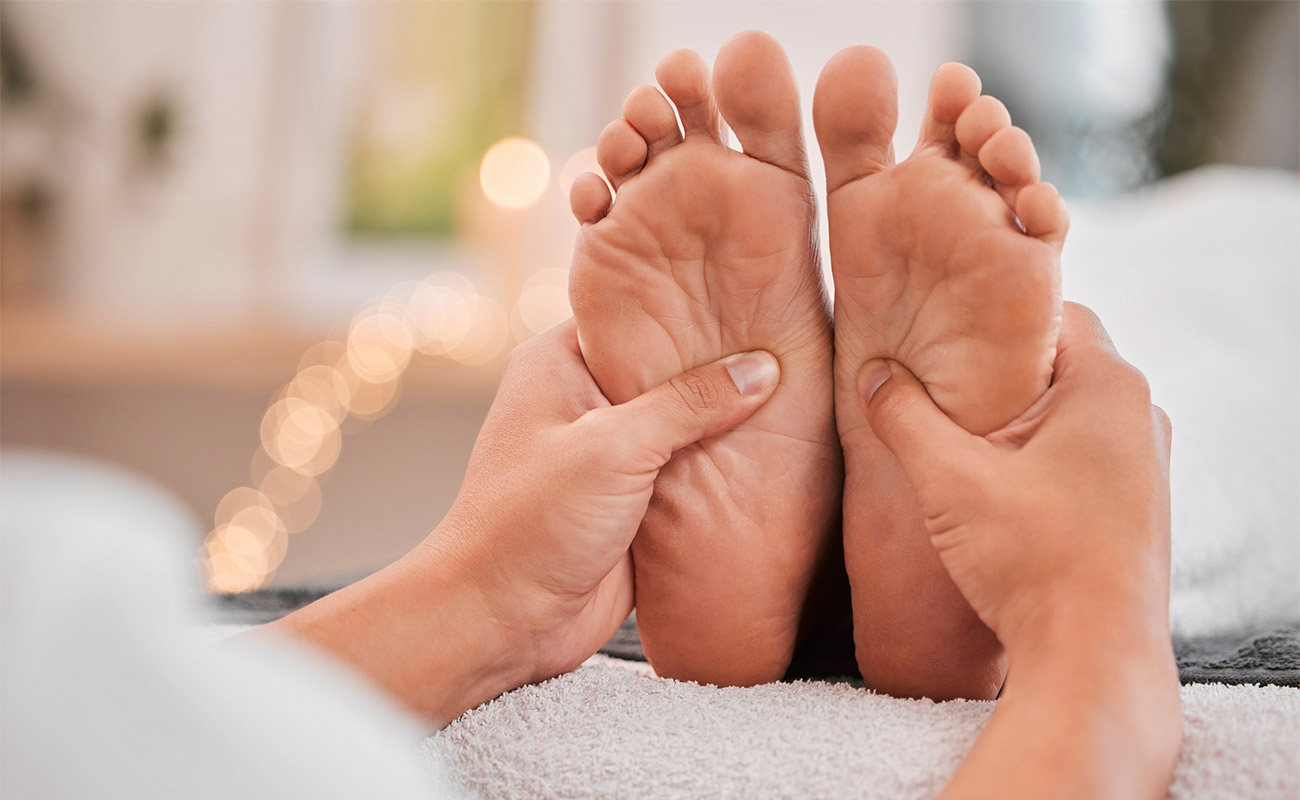This image is a detailed depiction of a therapeutic foot massage, likely intended to advertise massage services. At the center of the image are two feet pointing outwards toward the viewer, with a pair of hands skillfully pressing their thumbs into the soles of the feet, indicative of a massage technique. The feet and hands stand out sharply against the blurred background, drawing clear focus to the massage. Both individuals wear white clothing, characteristic of spa attire, which adds to the overall sense of cleanliness and relaxation. The feet rest on a white towel, creating a cohesive, serene aesthetic. Soft lights are visible in the background, enhancing the calming ambiance. The overall light and muted tones of the image, combined with the soothing context, contribute to a tranquil and inviting atmosphere.